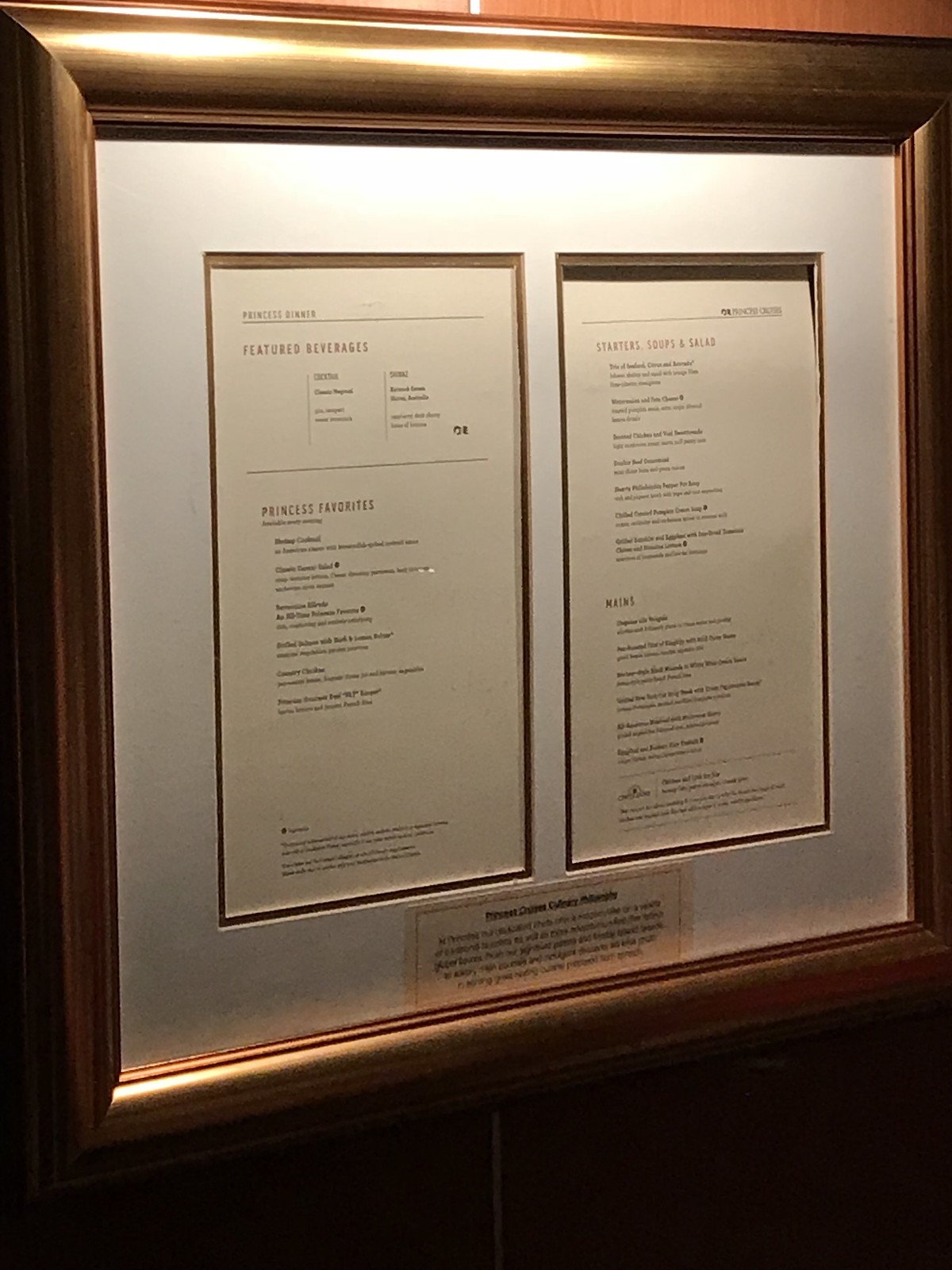The image depicts a framed menu mounted on a reddish-brown, wood-grained wall. In the upper right corner, the wall appears darker, creating a gradient effect. The menu frame is crafted from dark wood with a more pronounced brown than red hue. A white mat surrounds the menu, and beneath it, a hint of gold matting can be seen, adding a touch of elegance. 

The menu itself is divided into two sections. The left side is titled "Beverages" and features a list under "Princess Dinner Featured Beverages," followed by another section labeled "Princess Favorites" with six items listed. On the right side, the menu begins with "Starter, Soup, and Salad," listing seven options, and continues with "Mains," featuring another six dishes. 

Centrally placed between the two sections, there is a cream-colored plaque with brown writing, although the text is not legible. Additional writing is present at the bottom of both the left and right sides of the menu, likely describing details or ingredients of the dishes. This menu appears to outline various dinner options, showcasing a diverse selection for a special "Princess Dinner."